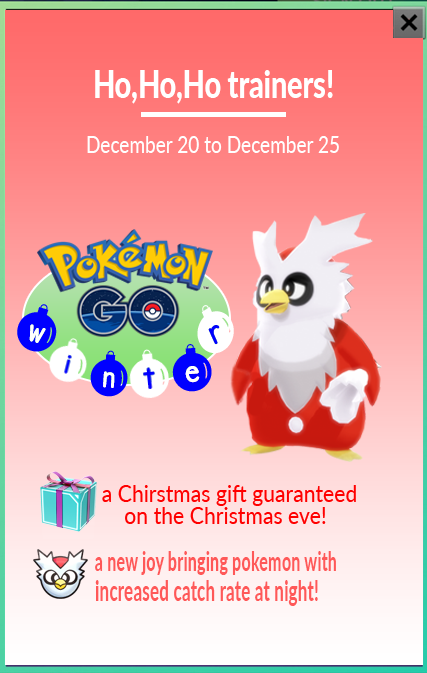The image features a rectangular box outlined in green. In the top right corner, there is a black "X" symbol. The background of the box transitions from deep red at the top, through pink, and nearly to white at the bottom. The text within the box reads, "Ho Ho Ho Trainers," followed by a line break, then "December 20th to 25th." Below that, the text says, "Pokemon Go Winter." 

Center of the image displays a whimsical bird-like Pokemon character with distinct features such as a white beard-like adornment and antler-like protrusions from its head. The character's eyes are black and white and appear cross-eyed. It wears a red suit with one white button and is holding an item tucked under its arm.

Further down, the text states, "A Christmas Gift Guaranteed on Christmas Eve," though "Christmas" is spelled incorrectly. There is an additional image of the same Pokemon character with a caption declaring it as "a new joy-bringing Pokemon with an increased catch rate at night."

This highly festive and detailed graphic seems to be promoting a special in-game event in Pokemon Go occurring from December 20th to 25th, emphasizing a guaranteed Christmas Eve gift and an enhanced ability to catch a particular Pokemon during nighttime.